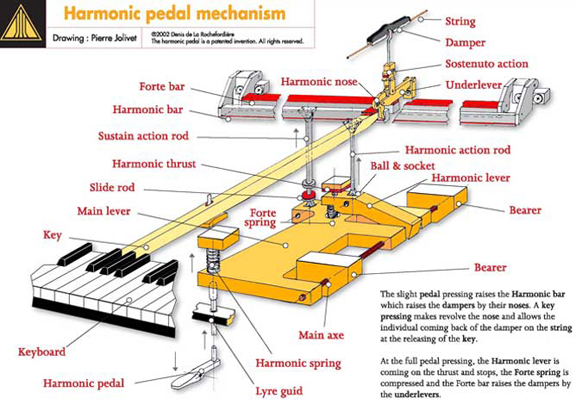This detailed schematic by Pierre Jolivet illustrates the intricate mechanisms of a harmonic pedal mechanism used in pianos. Set against a white background, the top left corner prominently displays the title "Harmonic Pedal Mechanism" in orange or yellow text beneath a pyramid-shaped icon on a black box. The image meticulously labels each component with red text, connected by dark lines to their respective parts, ensuring clarity. Key elements showcased include the string, damper, sun steno auction, under lever, harmonic action rod, ball and socket, harmonic lever, bearer, main axe, harmonic spring, lyre gid, harmonic pedal, keyboard, key, main lever, forte spring, side rod, harmonic thrust, sustain action rod, harmonic bar, and forte bar.

The majority of the diagram's base is yellow, featuring two prominent bright yellow rods at the top. A silver and red section capped with a black string sits at the uppermost part of the illustration. At the bottom right, a note explains that a slight pedal press raises the harmonic bar, detailing the functionality of these components. Additionally, on the left-hand side, there is a small black and white depiction of piano keys, correlating to the overarching piano structure.